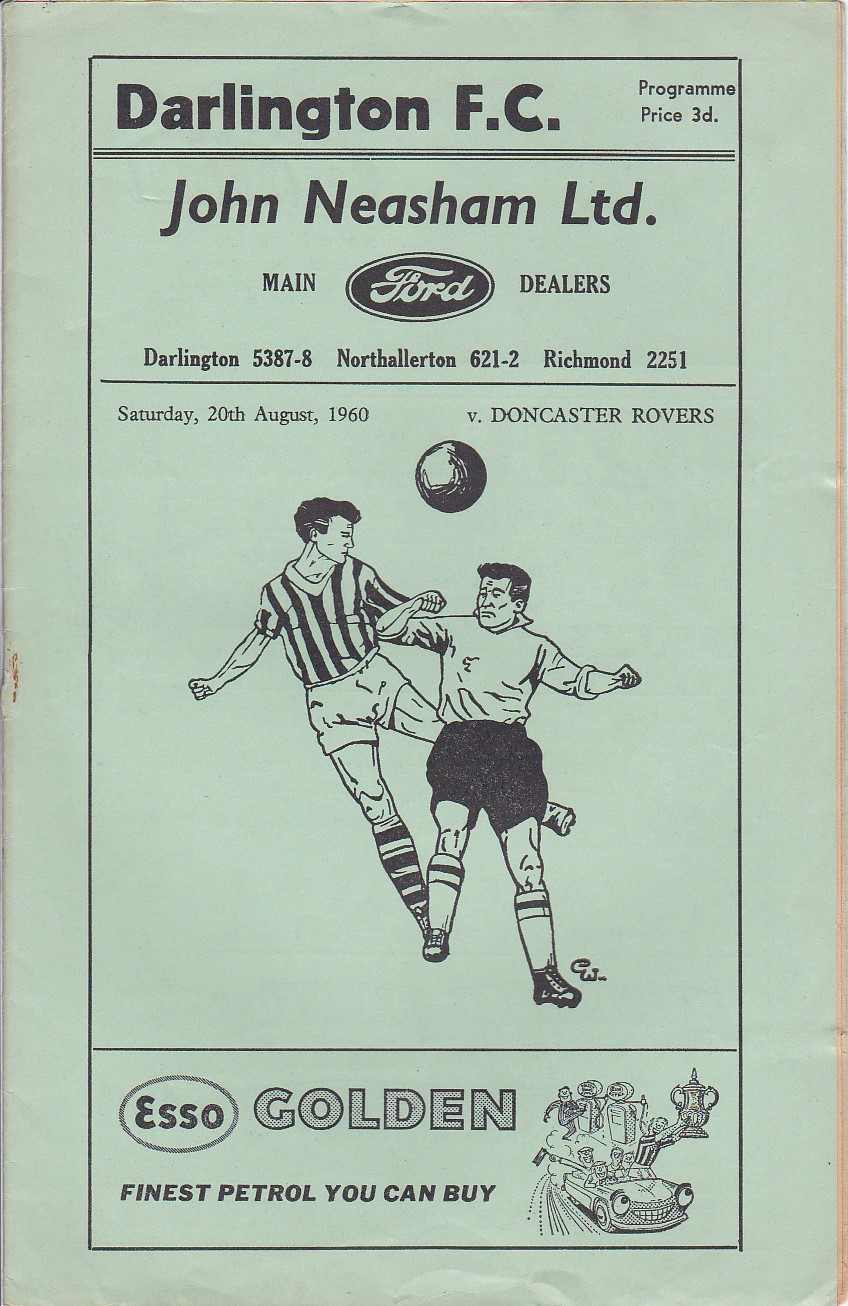This image showcases an antique program for a soccer match, specifically for Darlington FC versus Doncaster Rovers, dated Saturday, August 20th, 1960. The brochure has a worn, faded appearance, indicating its age, and was originally primarily green and black. Central to the design is a cartoonish pen drawing of two men engaged in a soccer action shot, one wearing a vertically striped shirt with matching socks, and the other in a plain white shirt with black shorts, with a soccer ball depicted above their heads. Above this, the program highlights an advertisement for John Neesham Ltd., the main Ford dealers, with the iconic Ford logo. It lists contact numbers for Darlington, North Allerton, and Richmond. The bottom of the brochure features an advertisement for Esso, promoting "Golden, the finest petrol you can buy" alongside a classic illustration of an old car. The program also notes that its price was 3D, emphasizing its vintage nature.